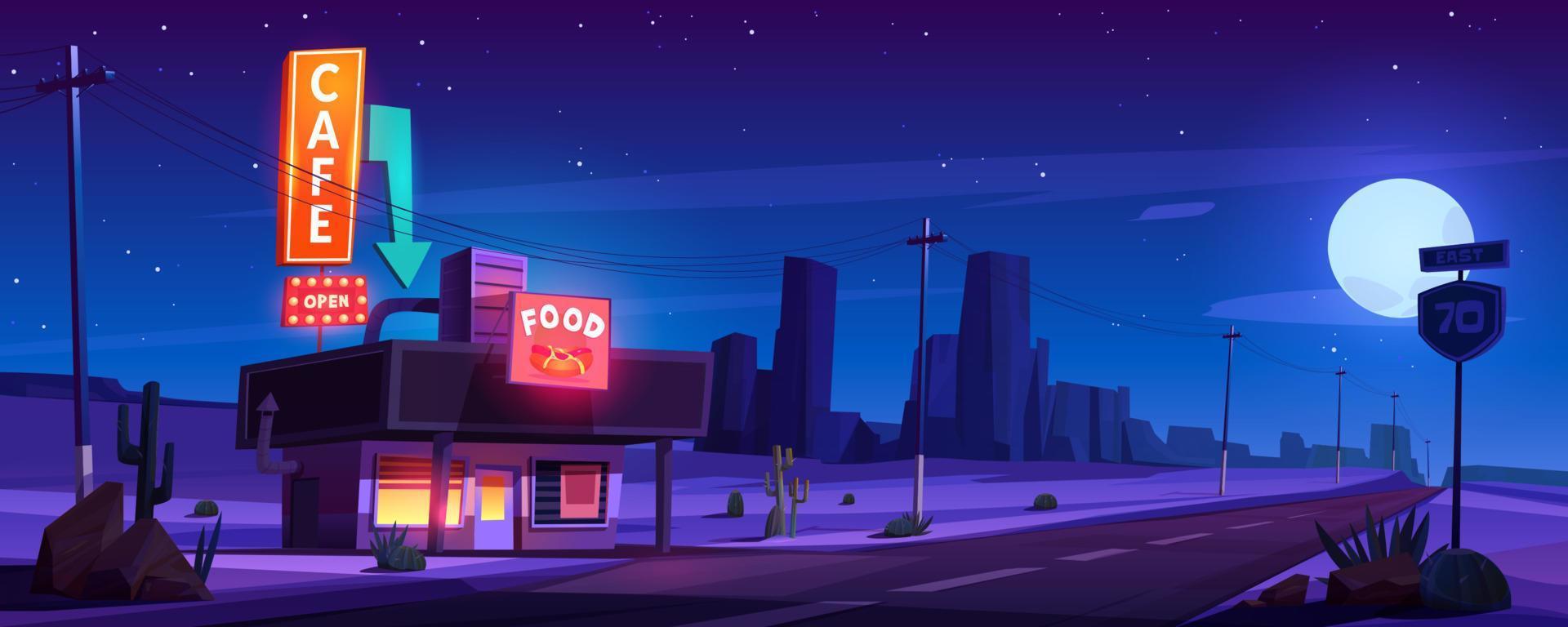In this detailed animated nighttime scene set in a desert, a small brick-and-mortar cafe stands illuminated along a highway. The ink-black sky, dotted with twinkling stars and a vibrant full moon, hints at the remote, serene location. Power lines stretch across the highway, guiding the viewer's eye to a sign indicating "East 70" and "Interstate 70" on the far right. Dominating the left-hand side, the cafe boasts bright orange and red neon signs reading "Cafe" with a blue downward-pointing arrow, and "Open" and "Food" alongside an appetizing depiction of a hot dog with mustard and ketchup. The glowing lights from within the cafe highlight its warmth and welcoming presence amidst the desolate desert landscape, complete with cacti and sandy terrain. Despite its isolated position, distant commercial skyscrapers subtly rise in the background, adding contrast and depth to the colorful, animated tableau.